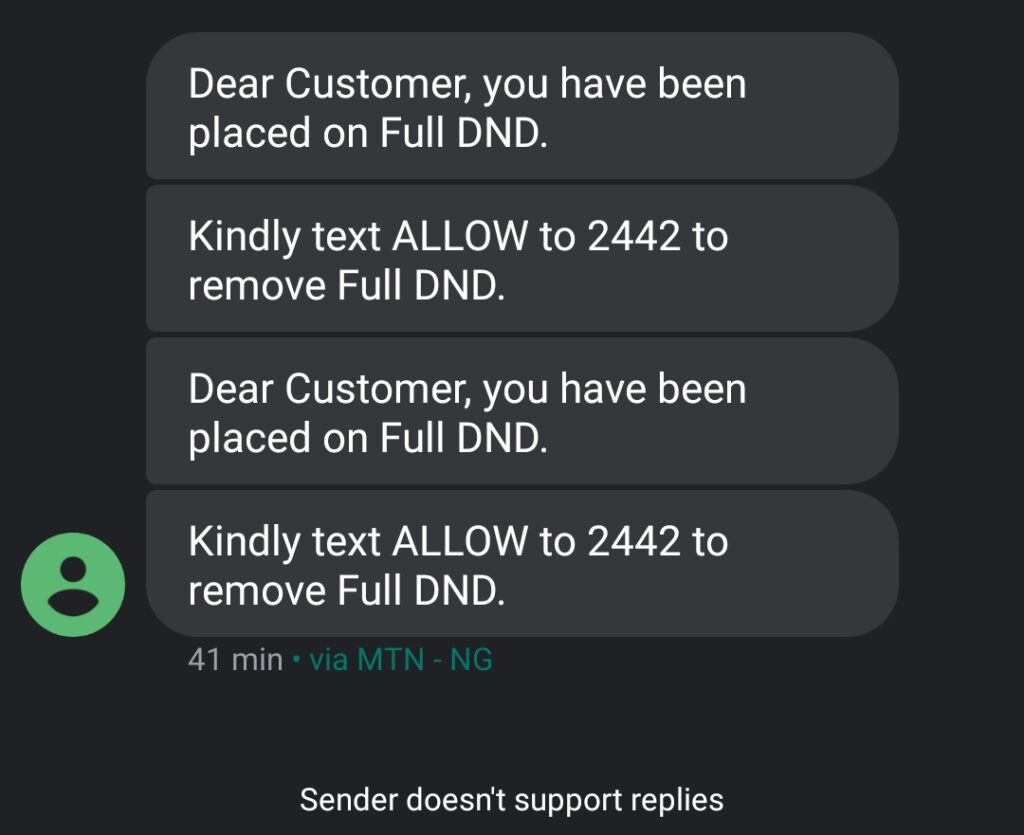This image features a partial screenshot of text messages displayed against a dark gray background. The backdrop is a sleek black box with a dark gray finish, enhancing the contrast with the white text. Four rounded rectangular text bubbles make up the core of the image, each containing the following messages:

1. "Dear Customer, you have been placed on full DND."
2. "Kindly text ALLOW to 2442 to remove full DND."
3. "Dear Customer, you have been placed on full DND."
4. "Kindly text ALLOW to 2442 to remove full DND."

The abbreviation "DND" (Do Not Disturb) is emphasized in capital letters in each message. Beneath these text bubbles, the note "41 Minutes, via MTN-NG" is written in green capital letters, indicating the time and the network provider. Accompanying this text on the left side is a small green icon depicting a bald-headed man with a collared shirt. The final line at the bottom of the image, written in white, states, "Sender doesn't support replies." This comprehensive view highlights the important details and formatting present in the screenshot.